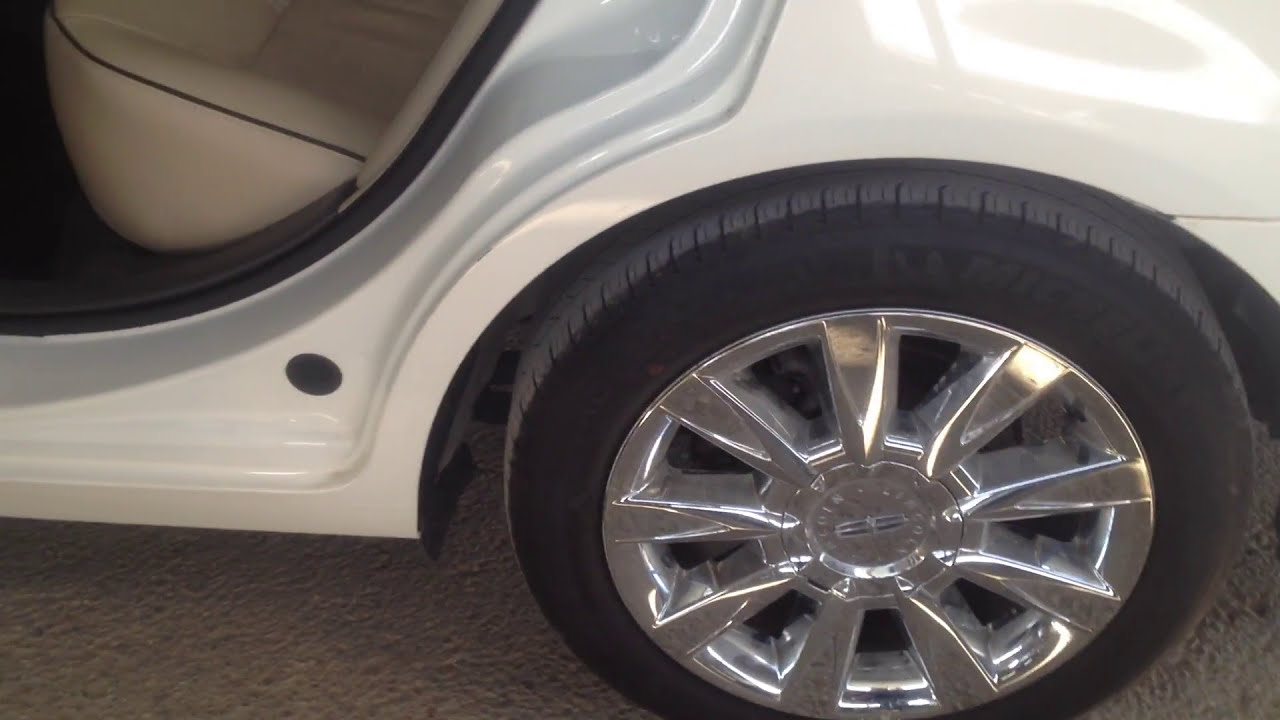The image showcases the left rear tire of a small white car on a tan and gray covered road. The prominently displayed tire is a Michelin with a significant amount of tread, mounted on a shiny chrome rim. The rim features the Lincoln insignia and logo centrally placed on the hubcap. The car’s rear quarter panel and rear passenger seat are noticeable, with the left side door open. Inside, the seats are upholstered in tan leather-like material with black lining, contrasting the dark gray or black flooring. Highlights can be seen on both the chrome wheel and the upper right corner of the image, enhancing the details of the vehicle's white exterior and beige interior. There is also a small black circle visible in the lower left corner of the picture.